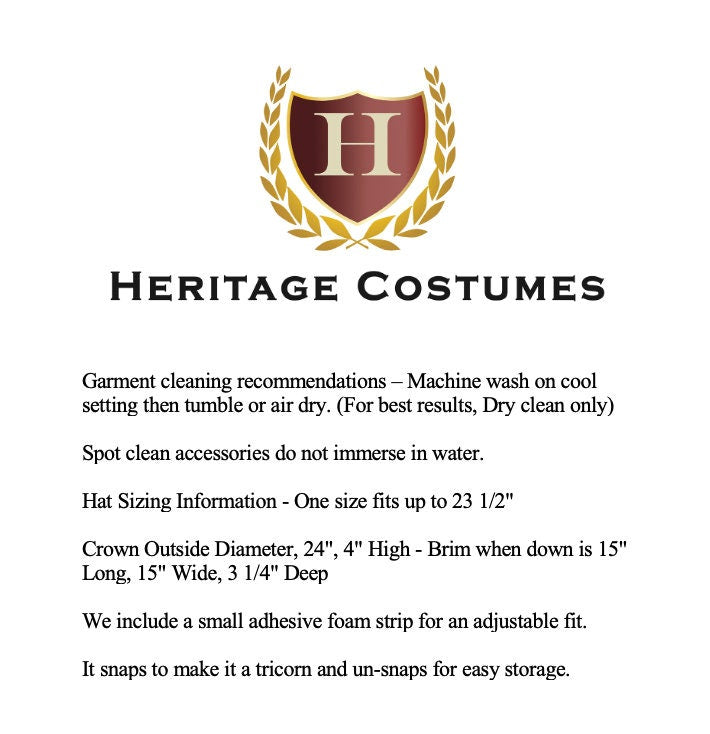Against a solid white background, the central image features a gold, U-shaped laurel leaf design reminiscent of ancient Roman motifs. Encased within the laurel is a dark brown shield adorned with a tan letter "H" at its center. Beneath the logo, bold black uppercase text reads "HERITAGE COSTUMES." 

Following this, smaller black text provides garment cleaning instructions: "Machine wash on a cool setting, then tumble or air dry. (For best results, dry clean only.) Spot clean accessories – do not immerse in water." 

Further down, the text details hat sizing information, stating, "One size fits up to 23 1/2 inches. Crown outside diameter: 24 inches, 4 inches high. Brim when down: 15 inches long, 15 inches wide, 3 1/4 inches deep." 

The description concludes with the note, "We include a small adhesive foam strip for an adjustable fit. It snaps to make it a tricorn and unsnaps for easy storage," emphasizing the practical design features and flexibility of the hat. The colors in the logo prominently feature gold, dark brown, and tan.